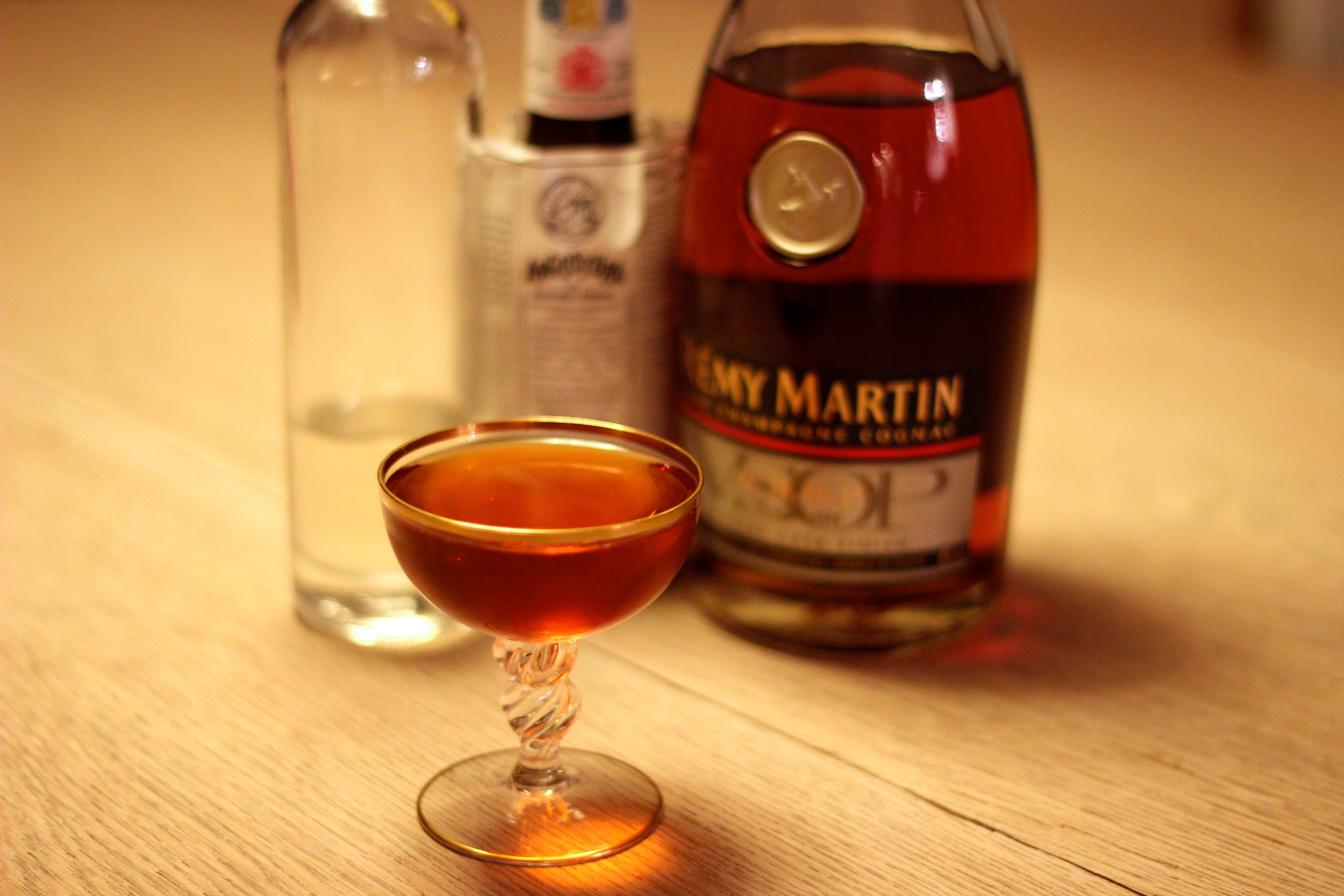The color photo is a close-up shot of a small glass of Remy Martin VSOP cognac. The glass is clear and adorned with a gold rim, and it is not a traditional cognac snifter but rather a very small round cup with a short glass stem. The cognac inside is a rich brown, almost golden color. In the background, an open bottle of Remy Martin VSOP cognac stands prominently. To its left, there's a slender, clear bottle with a transparent liquid, possibly water or vodka. To the right of the cognac bottle, there's a bottle with a blurred label, appearing shorter and smaller. All four items are placed on a light wood-grained table top surface, adding to the warm and inviting ambiance of the scene.